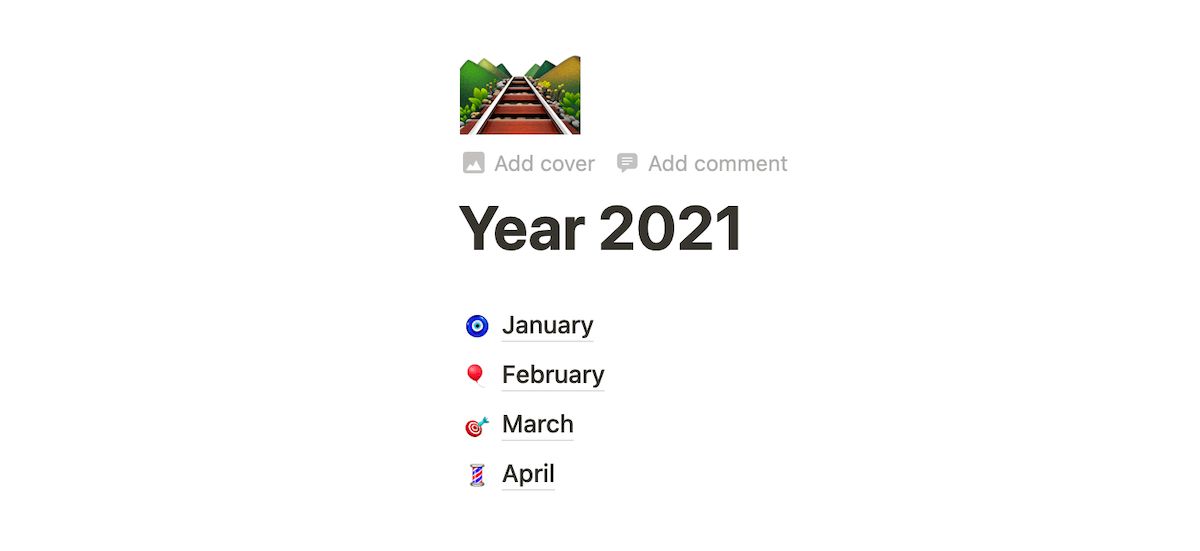In the image, the top left corner features a small profile icon depicting a railway track extending upwards towards the horizon. The metallic rails gleam in silver, supported by brown sleepers, while the ground on either side is dotted with brown and grey rocks. Flanking the railway are verdant mountains with patches of brown near the peaks. The landscape is dotted with green cactus plants and, on the right side, yellow flowers add a splash of color. Below the profile icon, grey text and icons indicate options to "Add Cover" and "Add Comment," with corresponding gallery and message icons. Beneath this section, the bold black text reads “Year 2021.” At the bottom of the image, months from January to April are listed in black text. January's icon comprises blue, white, light green, and black hues, while February features a red balloon. March is represented by a red and white target board, and April showcases a spherical object in blue, white, and grey.